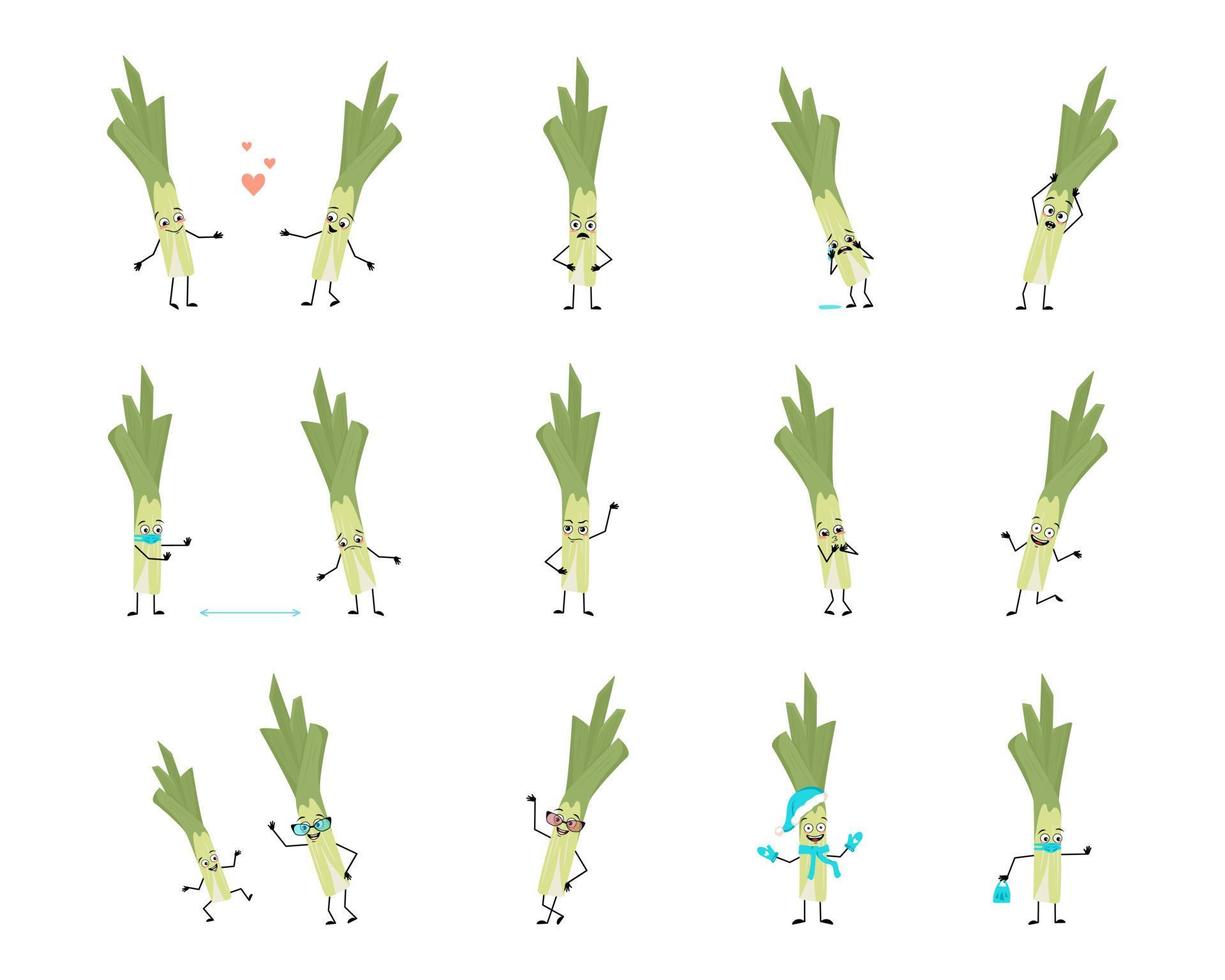The image is a detailed illustration of anthropomorphized asparagus figures, organized into three rows of five columns. Each asparagus character has a light green stalk for a body with darker green shoots sprouting from the top, resembling hair. They all feature expressive human-like faces with eyes, eyebrows, and mouths, along with small black stick arms and legs, complete with circular hands and feet.

In the first row, the characters exhibit a variety of emotions and activities: 
1. Two asparagus figures stand close, smiling at each other with three small red hearts between them.
2. A single, angry-looking asparagus with arms on its hips.
3. A sad asparagus, rubbing its eyes as if crying.
4. A surprised asparagus with its arms raised to its 'head'.
5. An asparagus celebrating, adorned in a blue and white Santa hat, mittens, and scarf.

The second row continues with diverse portrayals:
1. Two asparagus figures, one wearing a mask and gesturing to maintain distance, while the other frowns with an indifferent stance.
2. A lone asparagus with one hand on its hip, somewhat waving.
3. An asparagus figure with hands at its mouth in a gasp or shout.
4. A playful asparagus, dancing with one foot in the air and arms stretched out joyfully.
5. An asparagus holding a blue purse, complemented by pink sunglasses, waving with one hand on its hip.

The third row completes the set:
1. A dynamic duo with one little asparagus jumping energetically and another, likely an adult figure or parent wearing sunglasses, waving.
2. An asparagus with pink sunglasses, striking a confident pose with one hand on its hip and while waving.
3. Another festive asparagus with a blue stocking cap and scarf, looking cheerful.
4. An asparagus figure wearing a mask, holding a blue purse, and appearing to look toward the right.

Overall, each asparagus figure is uniquely personified, showcasing a wide range of emotions and accessories, vividly bringing the characters to life.